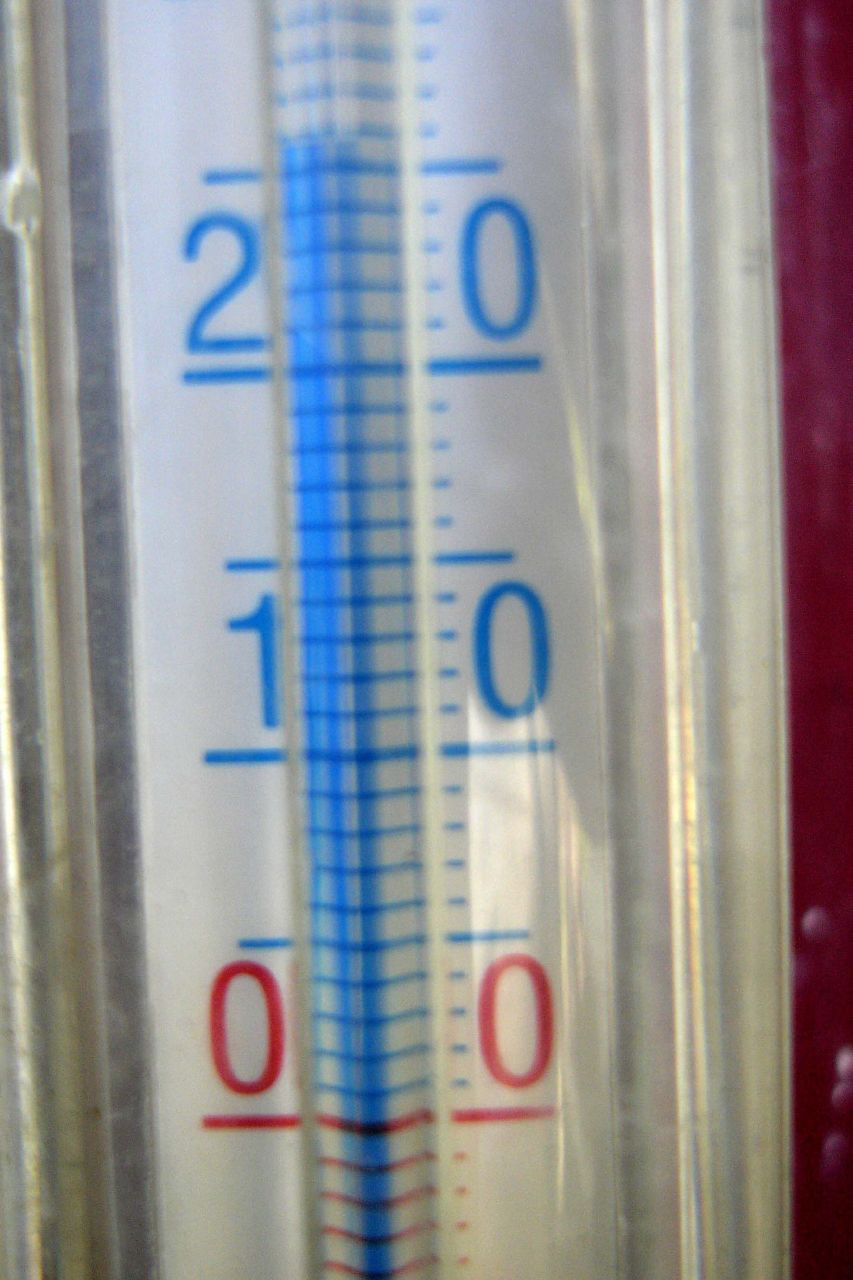This close-up photograph captures an intricate measuring instrument resembling a thermometer, prominently filling the frame from bottom to top. The backdrop on the far right is a deep maroon-red hue, which starkly contrasts with the transparent material of the gauge, seemingly made of plastic or glass. 

At the bottom of the thermometer-like device, five red horizontal lines are visible, with the topmost line being noticeably bolder. Just above this, the number zero appears on both sides of the gauge in a bright red color. 

Further up, blue vertical lines intersect the device, underlining a sequence of numbers. The first sequence features the numbers one on the left and zero on the right, marked in blue. These blue vertical lines continue upward, leading to the next sequence that displays the numbers two on the left and zero on the right, also in blue.

A prominent blue line runs vertically through the center of the gauge, extending upwards beyond the section containing the numbers two and zero. This detailed and meticulous design suggests that the instrument is designed for precise measurement, though the exact nature of what it measures remains ambiguous.